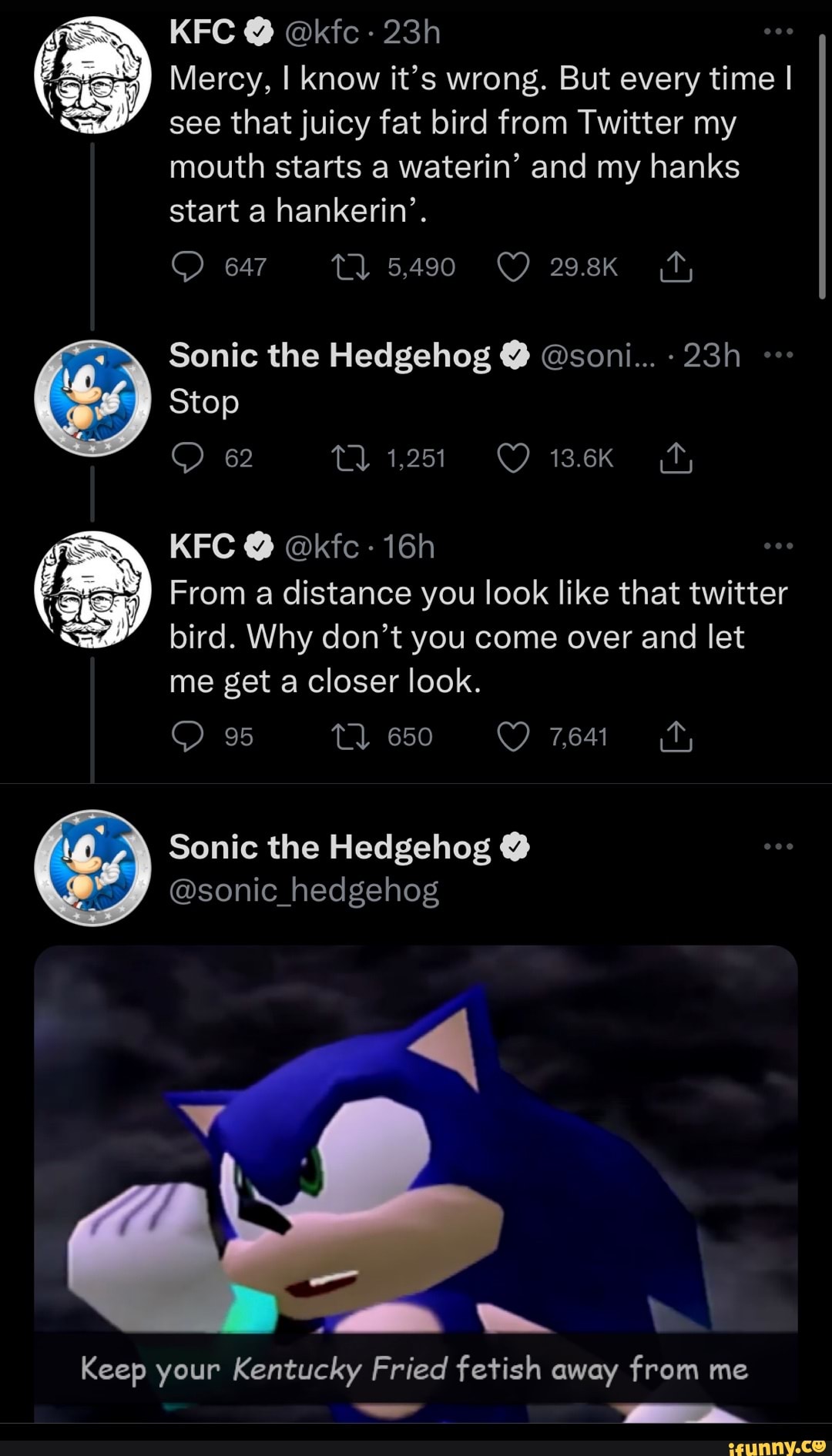This image is a mobile screenshot of a conversation on Twitter. The background is jet black, highlighting the exchange between the fast-food chain, KFC, and the iconic video game character, Sonic the Hedgehog. 

On the left, the KFC icon features a black-and-white depiction of Colonel Sanders. To the right of this icon, KFC initiates the dialogue: 
"Mercy, I know it's wrong, but every time I see that juicy fat bird from Twitter, my mouth starts a-waterin' and my hanks start a-hankerin'."

On the right, Sonic the Hedgehog's profile picture, a cartoon representation, responds succinctly: 
"Stop."

KFC continues, seemingly undeterred:
"From a distance, you look like that Twitter bird. Why don't you come over and let me get a closer look?"

At the bottom, Sonic retorts with an image showing him in an angry stance, his fist raised in front of his face. The text accompanying the image reads:
"Keep your Kentucky Fried fetish away from me."

In the bottom right corner of the screenshot, the watermark "ifunny.co" is visible. Below each message, light gray text indicates the number of comments, reshares, loves, and an upload button, common features of Twitter's user interface.